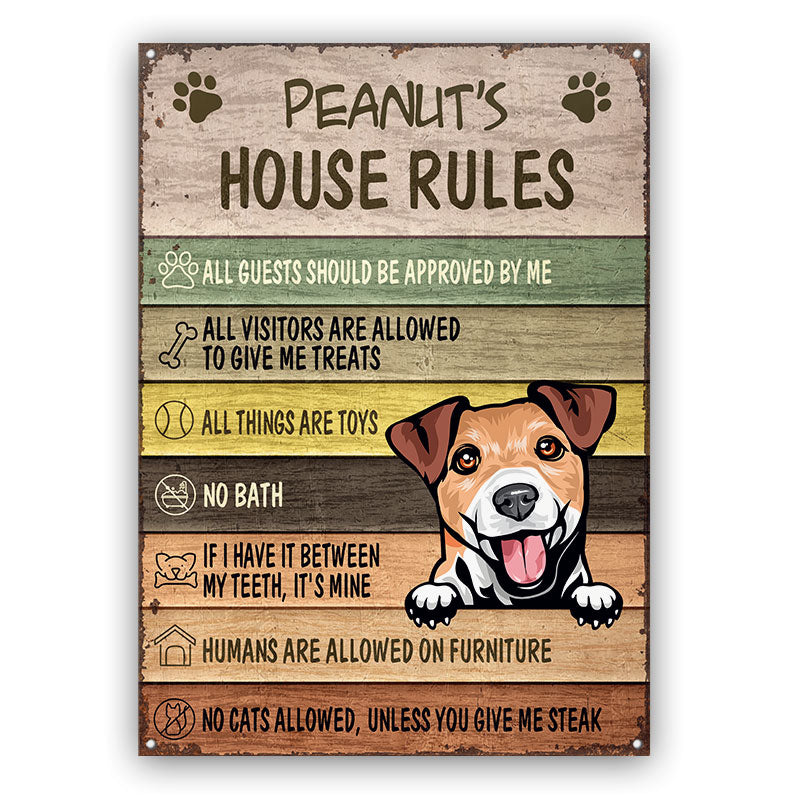This detailed description combines elements from each of the three provided captions with an emphasis on their shared and repeated details:

The image is of a decorative wooden wall plaque titled "Peanut's House Rules," featuring a rectangular design measuring approximately five inches high by three inches wide. The plaque is divided into eight horizontal sections, each bordered by thin brown lines. At the top, two small paw prints frame the title, written on a light brown background. Below, an illustration of a cheerful dog with floppy ears, a light brown face, dark brown ears, a white muzzle, and a big red tongue playfully hangs over the third section, giving the plaque a whimsical touch.

Each section of the plaque displays a humorous house rule from the dog's perspective, painted on different colored wood slats with matching images:
1. On a green background with a paw print: "All guests should be approved by me."
2. On a brown background with a bone: "All visitors are allowed to give me treats."
3. On a yellow background with a ball: "All things are toys."
4. On a dark brown background with a crossed-out bathtub: "No bath."
5. On a light brown background with a dog holding a bone: "If I have it between my teeth, it's mine."
6. On a brown background with a house: "Humans are allowed on furniture."
7. On a brown background with a crossed-out cat: "No cats allowed unless you give me steak."

The plaque has light gray circles at its corners for pinning onto the wall and features a light gray shadow effect around the border, giving it a framed appearance. The playful design and humorous rules make it a charming and comedic addition to any home.